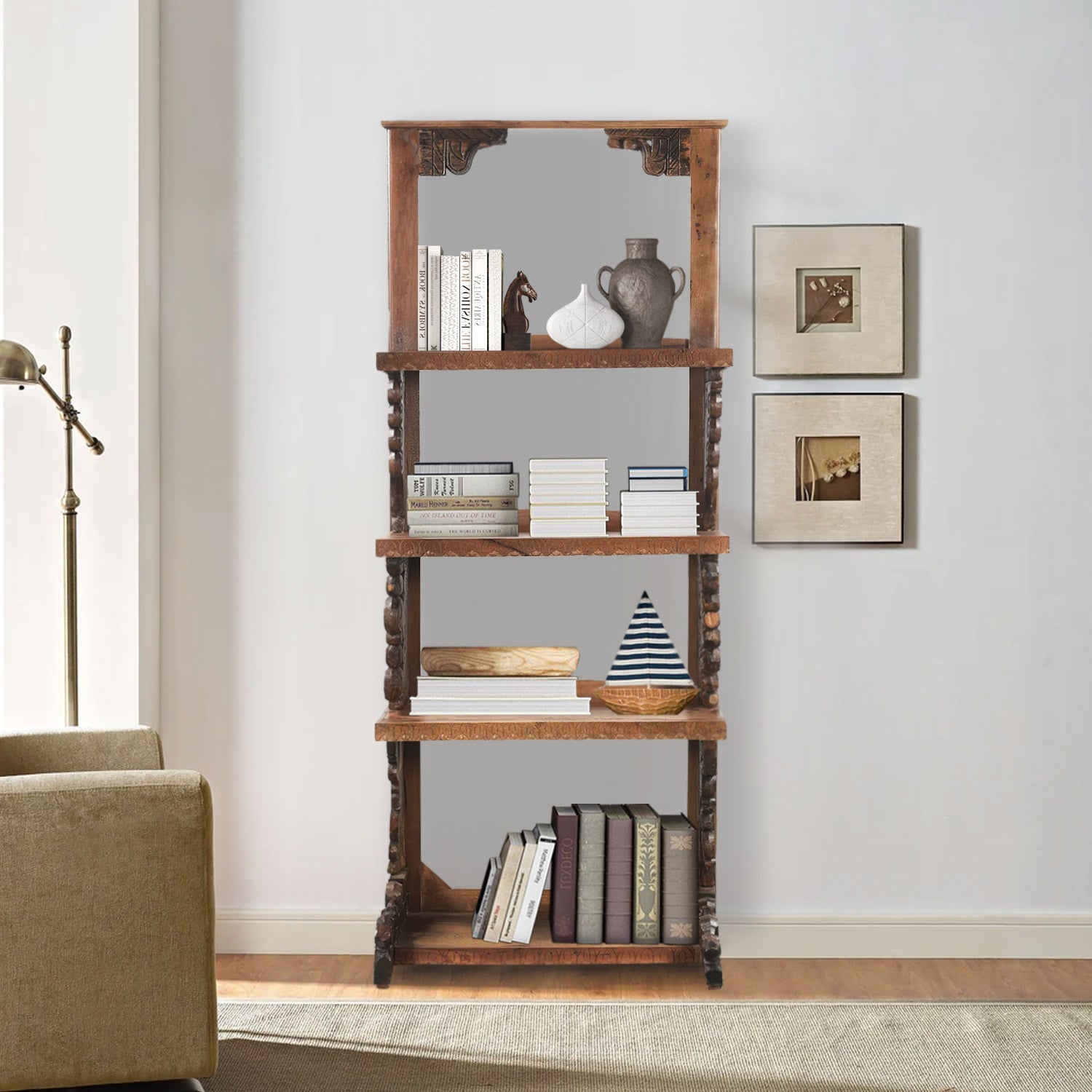In the image, an elegantly staged living room scene features a meticulously arranged set. Central to the composition is a five-tier wooden bookshelf, combining light brown and darker mahogany hues, set against a pristine white wall. The shelving unit stands on intricately detailed wooden legs and hosts an eclectic assortment of items. 

On the top shelf, a collection of books is accompanied by a gray vase, a white vase, a piece of pottery, and a dog-like ornament. The second shelf displays books stacked in various orientations, creating visual interest. The third shelf houses a charming wooden sailboat with a blue and white sail, flanked by more books. The bottom shelf contains an assortment of books, some neatly arranged while others lean casually against them. 

To the right of the bookshelf are two small picture frames with thick white borders, enclosing tiny, indistinct but artsy visuals. On the floor, a light tan runner carpet complements the wooden flooring. To the left, a beige upholstered chair, reminiscent of a recliner, nestles beside a modern yet timeless standing lamp, contributing to the overall cozy and sophisticated ambiance of the space.